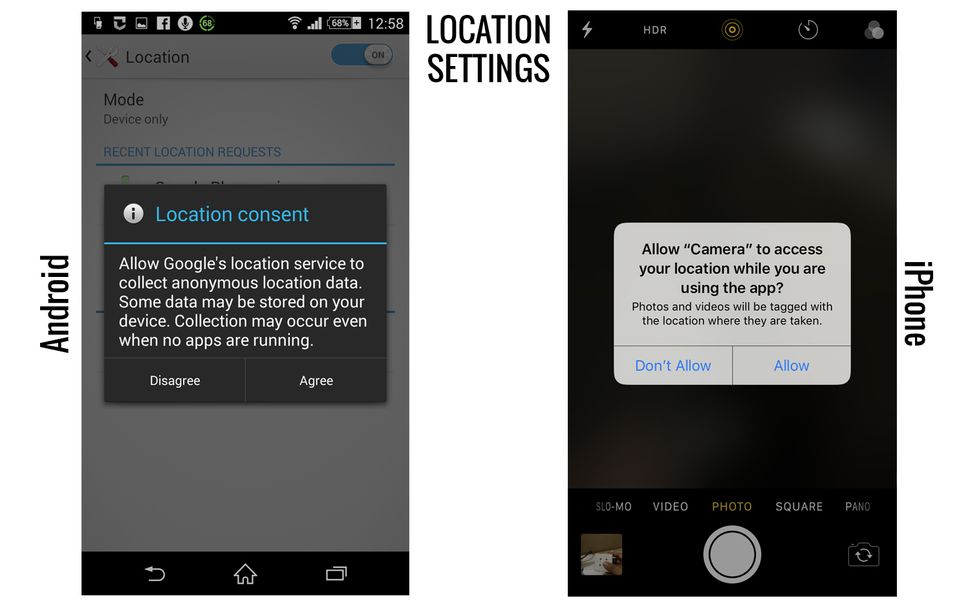Here is a detailed and cleaned-up caption for the image described:

---

The image displays two smartphone screenshots side by side, showcasing the location settings dialog on both an Android device (left) and an iPhone (right). The Android screenshot, with a black background and white text, prompts the user to grant location consent with the following message: "Allow Google's location service to collect anonymous location data. Some data may be stored on your device. Collection may occur even when no apps are running." Users can choose between "Disagree" or "Agree." The Android interface appears cluttered with several notifications at the top, including icons for Facebook, microphone, battery, Wi-Fi, data, another battery, screen sharing, and the time. In contrast, the iPhone screenshot, with a white background and black text, requests permission for the camera app to access the user's location, stating: "Allow camera to access your location while you are using the app. Photos and videos will be tagged with the location where they are taken." Users can choose between "Don't Allow" or "Allow." The iPhone's interface looks clean and free of additional notifications. 

---